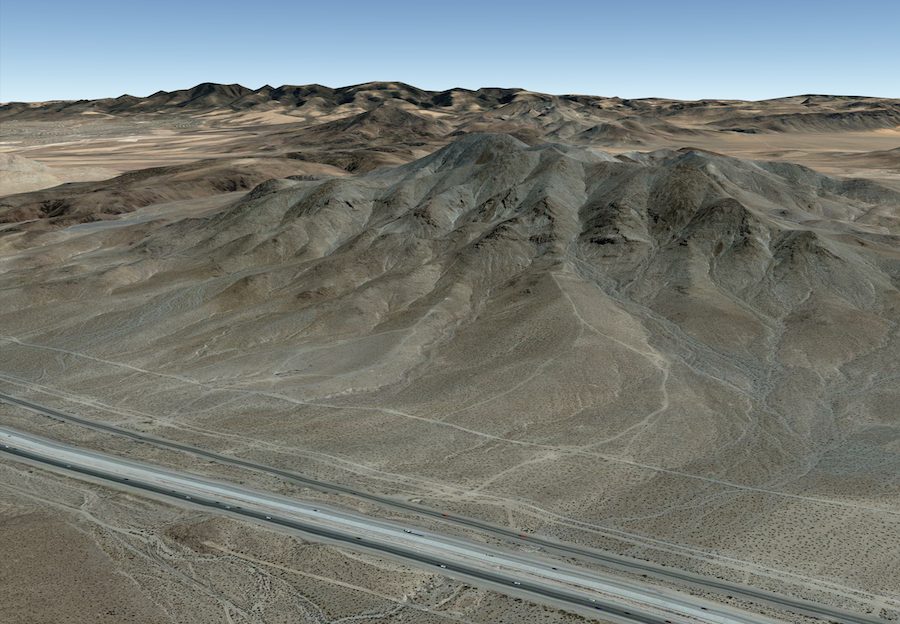This detailed photograph captures a desolate desert landscape taken from an aerial perspective. The foreground features a flat, black asphalt road that stretches from the lower left to the bottom right of the image, marked by lines indicating travel. On either side of the road, the terrain consists of beige, tan, and brown mountainous formations devoid of any vegetation. The colors in the scene are predominantly shades of gray, brown, and taupe, with the only additional color being the light blue, cloudless sky in the background. Dots, possibly cars, are visible along the highway, enhancing the sense of scale in this otherwise barren and dry environment. The stark absence of trees, grass, flowers, or water emphasizes the harsh, barren nature of the desert landscape.